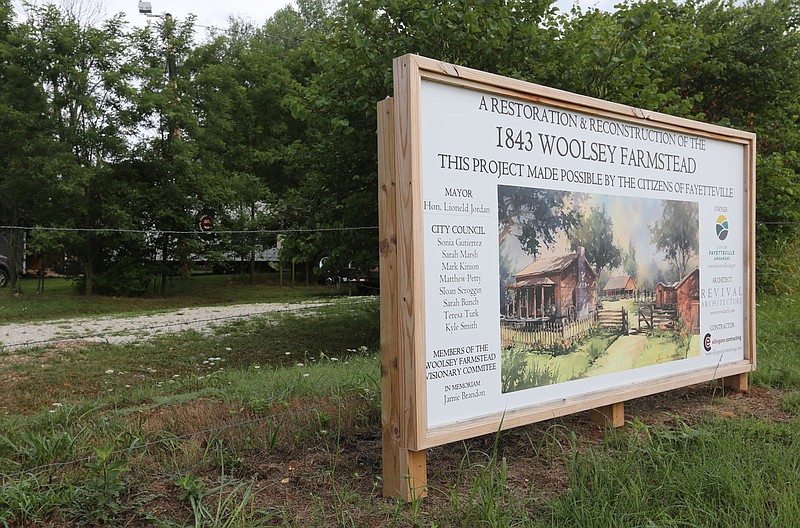This color landscape photograph captures an outdoor scene featuring a wooden-framed sign situated in a field of long grass interspersed with patches of brown, weeds, and white flowers. The sign, positioned close to the ground on short, protruding posts, is a horizontal rectangular shape with a light pine-colored frame. The white panel of the sign prominently displays the text: "A restoration and reconstruction of the 1843 Woolsey farmstead. This project made possible by the citizens of Fayetteville," written in large black letters at the top. Below this, a color illustration depicts an old log cabin site with wooden houses, grass, trees, and wooden gates. To the left of the illustration, the sign lists the names of Mayor Honorable Lionel Jordan and city council members, while the right side features sponsor logos, though some smaller text is blurry. The background includes a fence to the left, contributing to the scene's photographic representationalism and realism with a blend of color illustration.